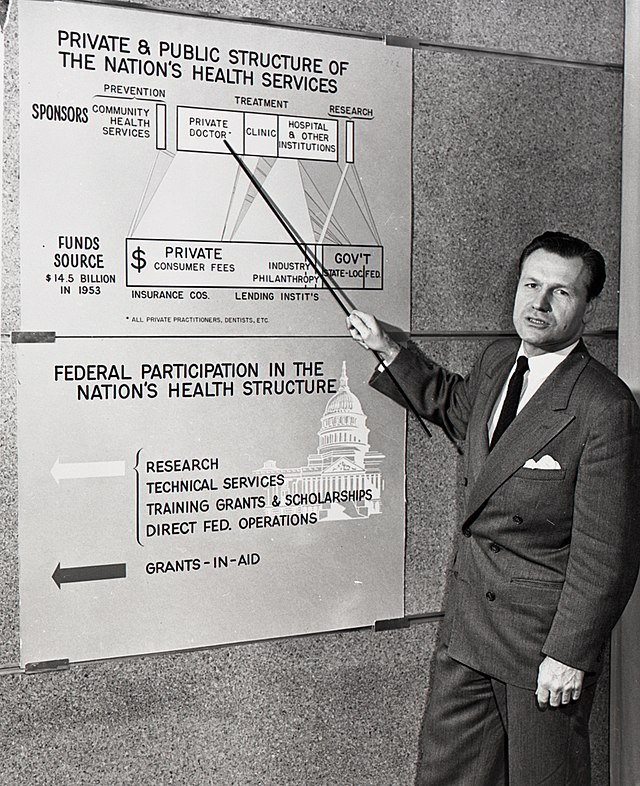The black-and-white photograph, oriented vertically, captures a formally dressed man presenting information on a wall-mounted poster. The man, with fair skin, dark eyes, and short dark hair, is dressed in a distinguished manner, wearing a crisp white shirt complemented by a solid dark tie and a double-breasted dark suit adorned with a white pocket square. He appears to be directly engaging the viewer or the photographer with a composed expression while holding a long, dark-colored pointer in his right hand, gesturing towards the poster to his left.

The prominently featured poster is divided into multiple sections and begins with the title, "Private and Public Structure of the Nation's Health Services." Following this, the headings "Prevention," "Treatment," and "Research" organize the poster's content. A detailed chart under the "Treatment" section lists various components that include private doctors, clinics, hospitals, and other institutions, visually explaining the diverse elements involved in healthcare delivery.

The lower portion of the poster is titled, "Federal Participation in the Nation's Health Structure," and includes an image of the Capitol building as part of its design, insinuating the governance and oversight role in healthcare services. The man's precise and authoritative stance, coupled with his professional attire and the informative poster, suggests a formal presentation or educational session focused on the complexities of the nation's health services infrastructure.